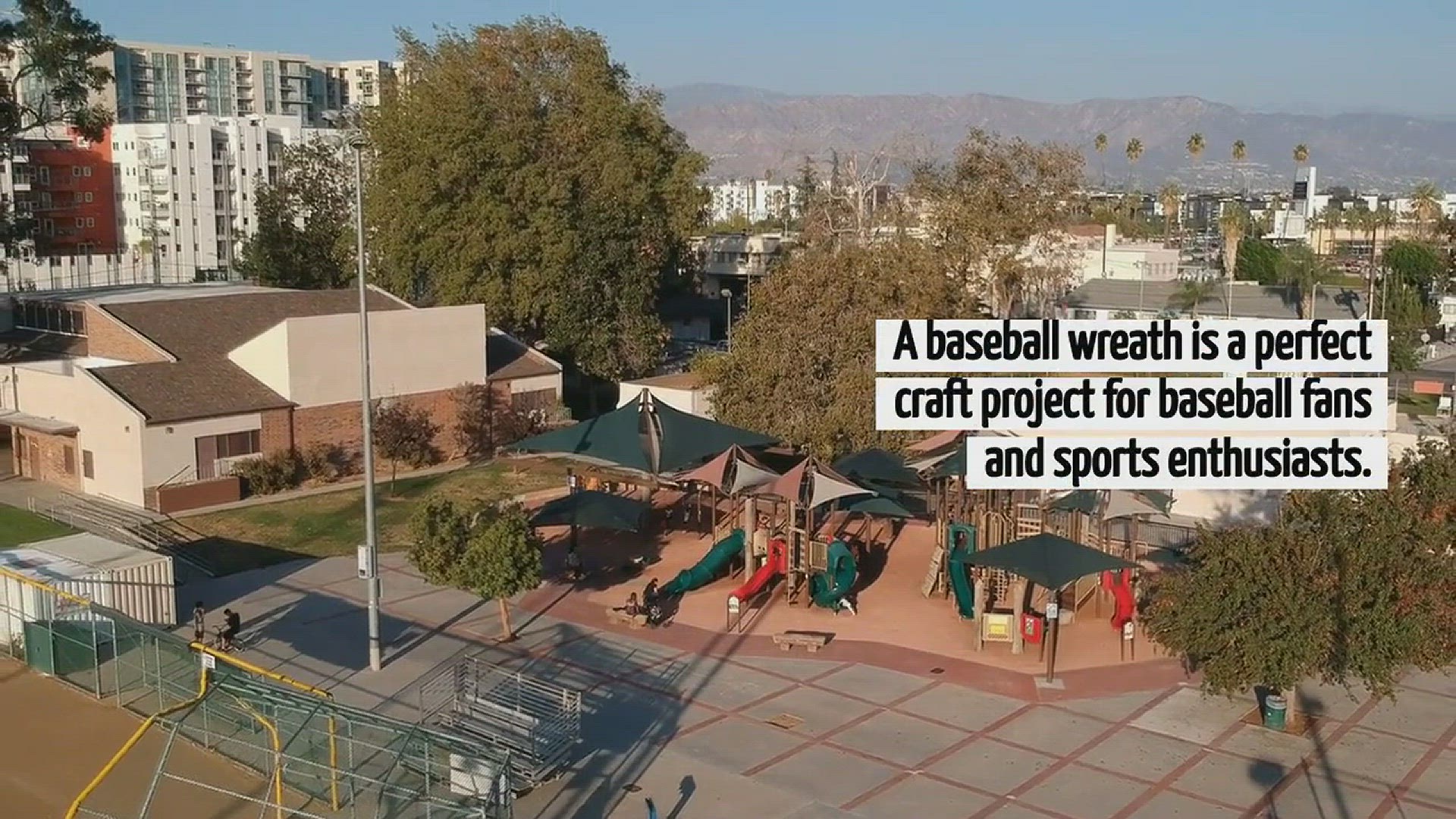This overhead photo showcases a bustling city park, believed to be in a Californian city such as Los Angeles or perhaps the Bay Area, encircled by numerous buildings and palm trees. Dominating the center of the park, there is a paved area with large gray tiles, featuring several large umbrellas providing shade. The image highlights two or three playgrounds, equipped with slides, scattered amongst a few trees. On the bottom left, a sports field, possibly a baseball field, is visible, marked by a sandy area. Nearby, a large brick building, potentially affiliated with the park or a recreational center, stands out. In the background, white buildings with windows and balconies as well as some rolling hills are visible. In black text across the top of the image, the words "a baseball wreath is a perfect craft project for baseball fans and sports enthusiasts" are somewhat incongruently displayed. Additional details include a recycling can near the center and another building situated on the top right corner of the image.